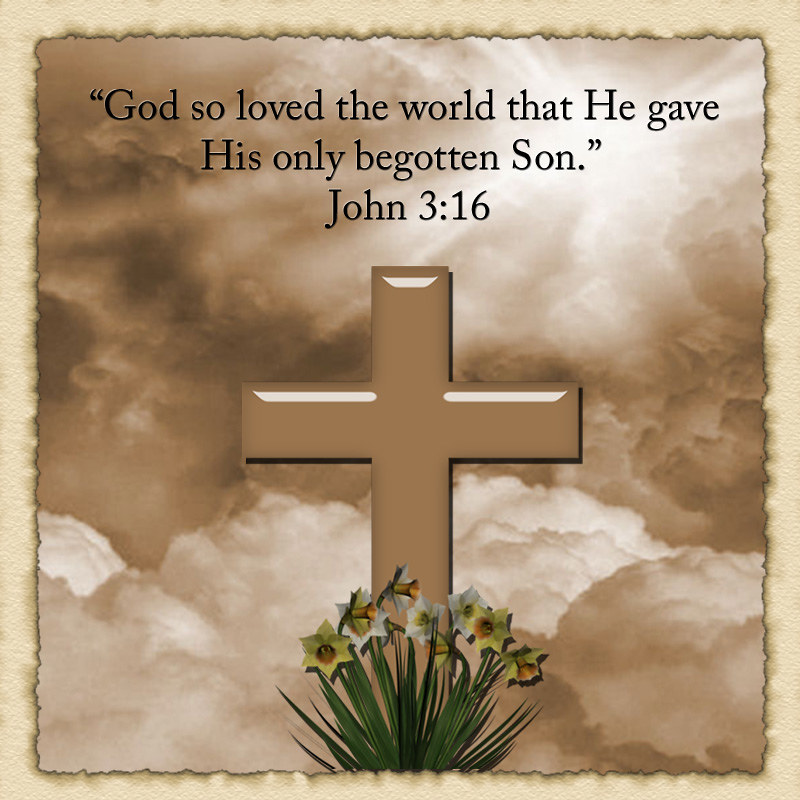The image features a square graphic with a tan, cream-colored base layer. Overlaid on the first square is a second square with jagged, burnt-paper-like edges and a black drop shadow. The central square portrays a sepia-toned scene resembling clouds with a beam of light descending from the top right. In the middle of this scene stands a brown, glossy, beveled cross, with yellow and white daffodils growing at its base. Centered above the cross, both horizontally and vertically, is the Bible verse John 3:16, which reads, "God so loved the world that he gave his only begotten son," in quotation marks. The overall design appears to be the result of an amateur graphic design project.